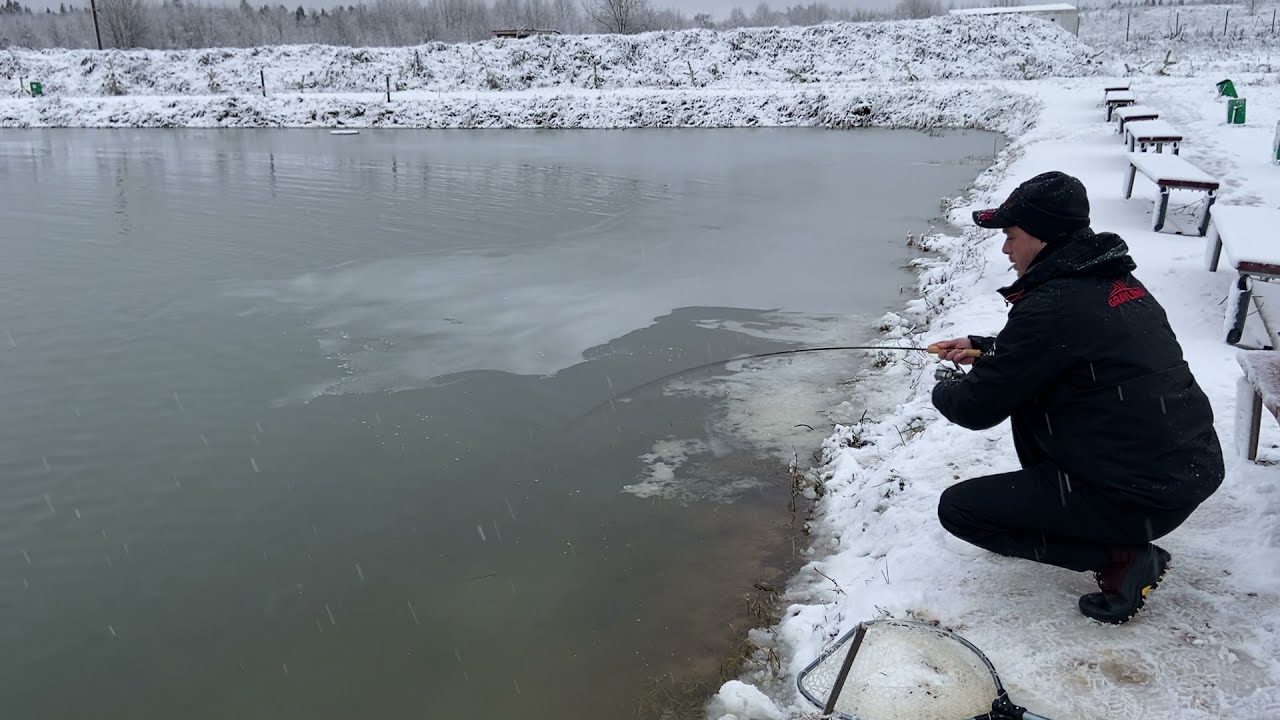This image captures a detailed scene of a man ice fishing by a rectangular, snow-bordered pond or lake under a cloudy, gray sky. The man is dressed in a black ensemble, including black boots, pants, a jacket with a red logo reading "Grayling," and a black hat with a red accent. He's crouching near the water's edge, holding a thin fishing pole that bends downward, suggesting he might have caught something. A steel net lies beside him, prepared for any catch. The water appears dark gray with hints of green, partially frozen at the top right corner.

The setting is starkly wintery, with snow blanketing the ground, nearby benches, and distant trees. These green benches line the right side of the image, stretching towards the back and covered in layers of snow. Footprints mark the snow around the man, indicating recent activity. In the background, a snow-patched wall is visible, adding to the structured feel of the setting. Green trash cans and a building can be seen further away, immersing the scene in a solitary yet tranquil winter landscape.